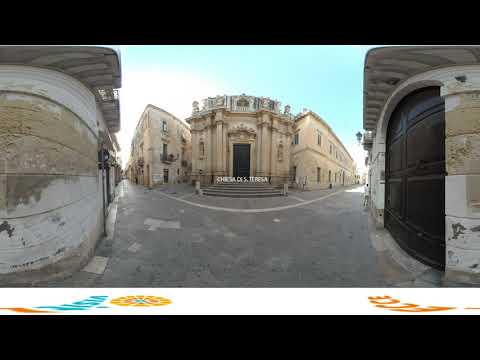In the center of the image, there stands a grand tan-colored building resembling a medieval church, adorned with ornate crown moldings and intricate designs on its flat roof. The building features a prominent dark-colored door, accessible by several white, wide steps leading up to it. Flanking this central building on both left and right are additional tan buildings with aged, flaking paint, contributing to an old-timey Mediterranean ambiance reminiscent of Italy. To the far left, there's a bulging, rounded structure in tan and beige hues. On the right, there's a similarly bulging structure with a dark-colored inset resembling a large garage door. The setting appears to be a quiet, light-flooded town road with no visible sky details due to the overpowering daylight, and devoid of people or cars, presenting an atmosphere of serene antiquity.